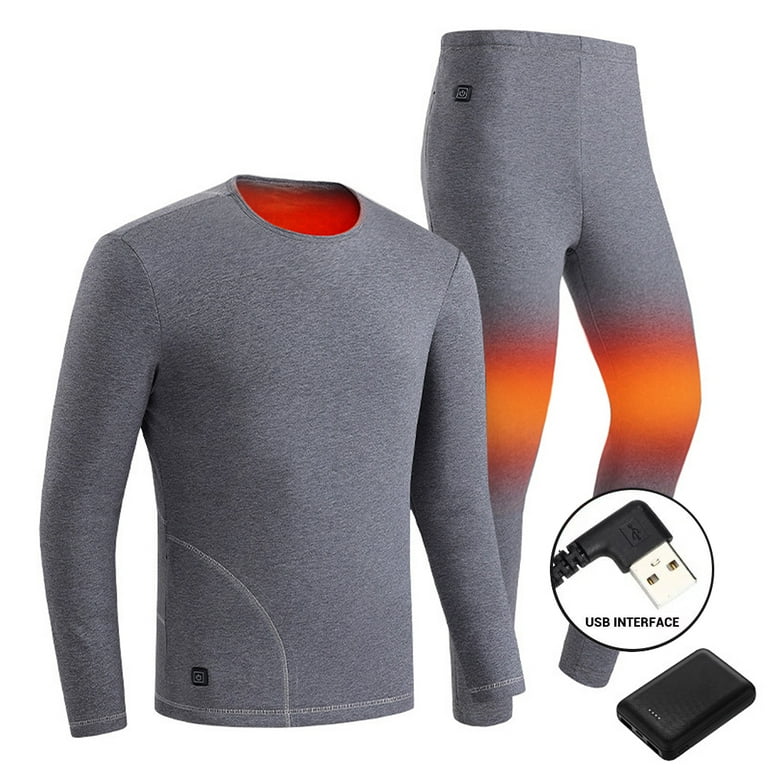This is a detailed product photograph showcasing a coordinated set of gray athleisure wear consisting of a long-sleeved shirt and leggings. The garments are crafted from a material resembling cotton or polyester, featuring intricate stitching details. The shirt has an orange lining inside the neck, while the leggings have orange-red markings around the knees, possibly indicating heated zones. Additionally, the image includes a small, black device with rounded corners, reminiscent of an old pager, connected via a USB interface. This device is likely a battery pack designed to heat the designated areas of the apparel, making it ideal for keeping the wearer warm in cold outdoor conditions or during leisurely activities.